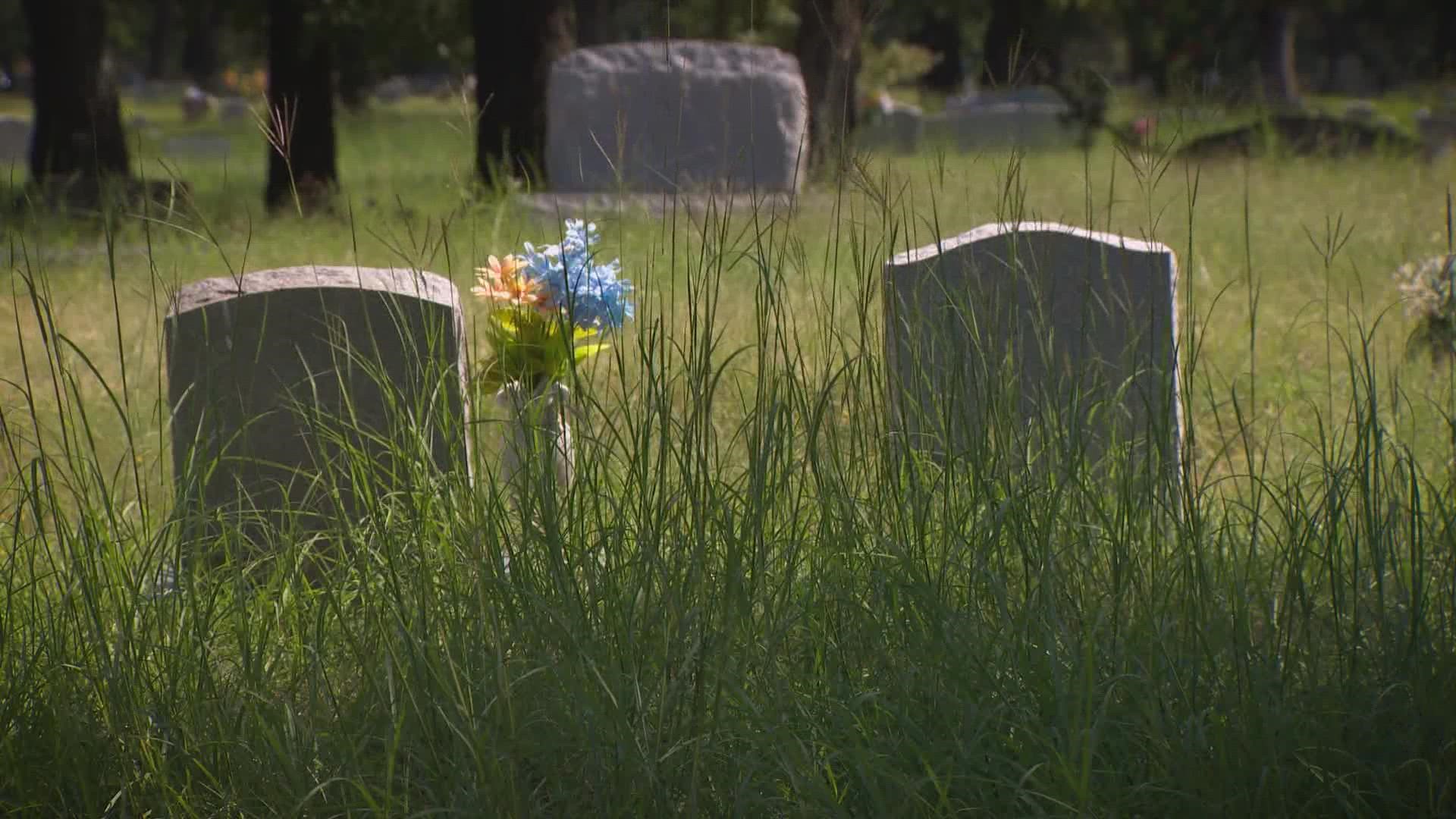The image captures an overgrown cemetery with a focus on two prominent gravestones in the foreground. These stones are partly obscured by tall, unkempt grasses that suggest the area has not been mowed or maintained for quite some time. The gravestone on the left is accompanied by a vase containing fresh flowers, including vibrant orange and blue blooms, standing tall beside it. The gravestone on the right is without flowers. Both stones are about two feet tall, solid, and vertical, with no visible inscriptions. Behind these stones, the canopy of trees and additional gravestones can be seen, but they are blurred and less distinct, giving the image a solemn atmosphere. The color palette predominantly consists of greens from the grass and trees and grays from the tombstones, creating a stark contrast with the colorful flowers. The photograph is taken from a low angle, emphasizing the neglected state of this section of the cemetery, while hinting at better-maintained areas in the distant background.